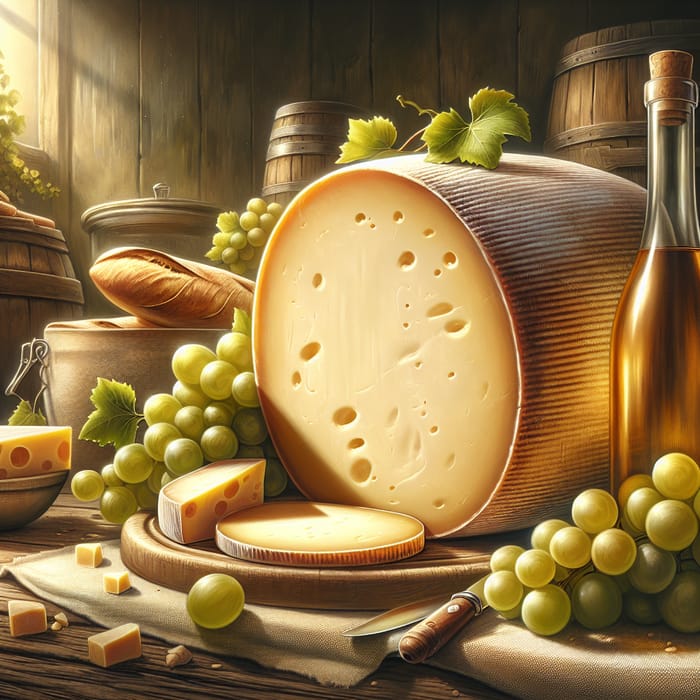The image appears to be a highly detailed and realistic representation, possibly AI-generated, capturing the rustic charm reminiscent of a Vermeer painting. At the center is an extensive, oval-shaped wheel of cheese, partially sliced to reveal large, bubble-formed holes, suggesting it may be Swiss cheese. Surrounding this focal cheese wheel are scattered green grapes and grape leaves, some of which drape over the cheese itself. Complementing the setting, there are two cheese knives and several cut pieces of cheese displayed with precision. A pot containing a baguette sits to the left, adding texture to the scene, while in the background, barrels suggestive of wine or rum storage enhance the rustic ambiance. There's also a glass bottle with a golden liquid—potentially olive oil or mead—with an elongated neck and cork. The sideways illumination from a window in the top left bathes the scene in soft, realistic light, creating a timeless, old-fashioned atmosphere.